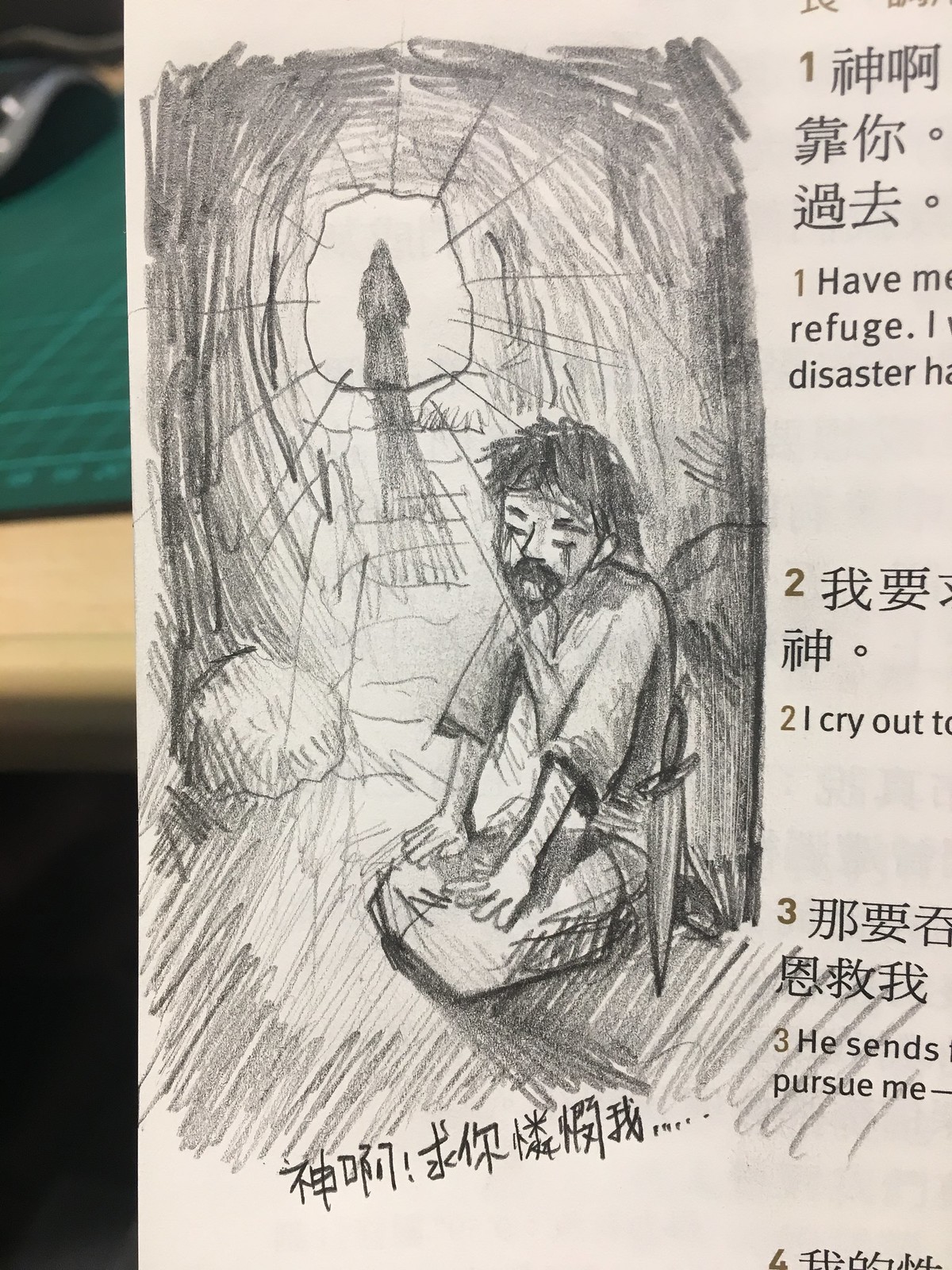An intricately detailed drawing occupies most of a white piece of paper positioned in photographic portrait mode. On the left edge of the image, there's a vertical band consisting of various textures and colors—mentioning from bottom to top: a dark shadow, a light wood floor, a patch of green that might be a carpet, and a section of black at the top.

The central focus of the drawing is a man depicted kneeling solemnly in front of what seems to be a lantern or an open flame. The man is dressed in attire evocative of traditional Asian garments, with a sword securely fastened by his side, adding to the sense of ancient custom and ritual. At the lower part of the artwork, a series of Chinese or Japanese characters is elegantly inscribed, while supplementary text in both Japanese and English is visible on the right side. The combined elements provide a rich, cultural narrative and convey a profound sense of purpose and tradition.